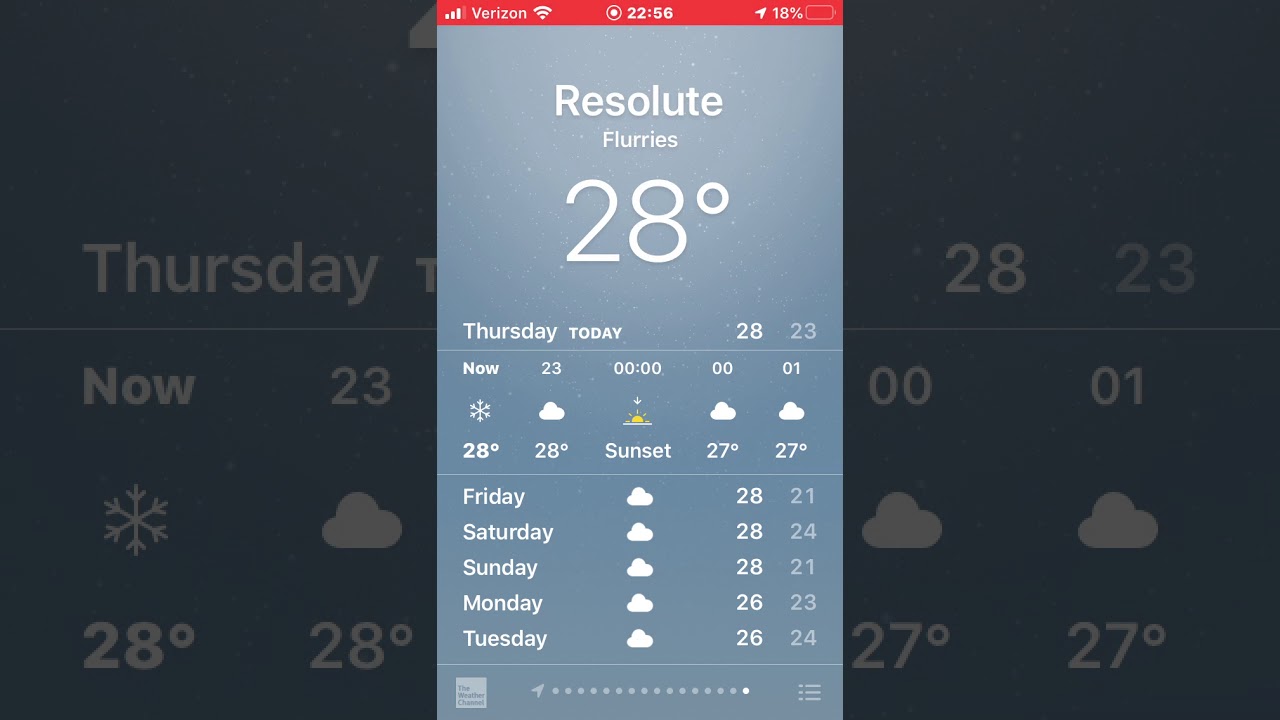The image features a grayed-out background displaying a weather interface partially obscured by a pop-up window. The background shows the day "Thursday" in white font, accompanied by temperature details. The visible information includes the temperature "now" as 23°C and various weather icons such as a snowflake and cloud symbols suggesting different weather conditions. Additional temperatures listed are "28, 23, 28, 27, 27".

The overlaying pop-up appears to be a screenshot taken from a mobile device. At the top of the screenshot, a red banner indicates "Verizon" with three signal bars, a Wi-Fi symbol, the time "22:56", and a battery indicator at 18%. Also visible is a small paper plane icon, typically representing message sent notifications.

The body of the pop-up specifies the location "Resolute" with the current weather condition as "flurries" and a temperature of 28°C. Below, it mentions "Thursday today" with similar temperature readings of 28°C. An icon for sunset is present, colored gold and white, with further temperatures listed as 27°C.

At the bottom section of the pop-up, the high and low temperatures for the upcoming days are detailed alongside cloud icons:
- Friday: 28°C / 21°C
- Saturday: 28°C / 24°C
- Sunday: 28°C / 21°C
- Monday: 26°C / 23°C
- Tuesday: 26°C / 24°C

The image concludes with a weather channel logo at the bottom, surrounded by various icons including a series of circles, a paper plane icon, and a list icon.